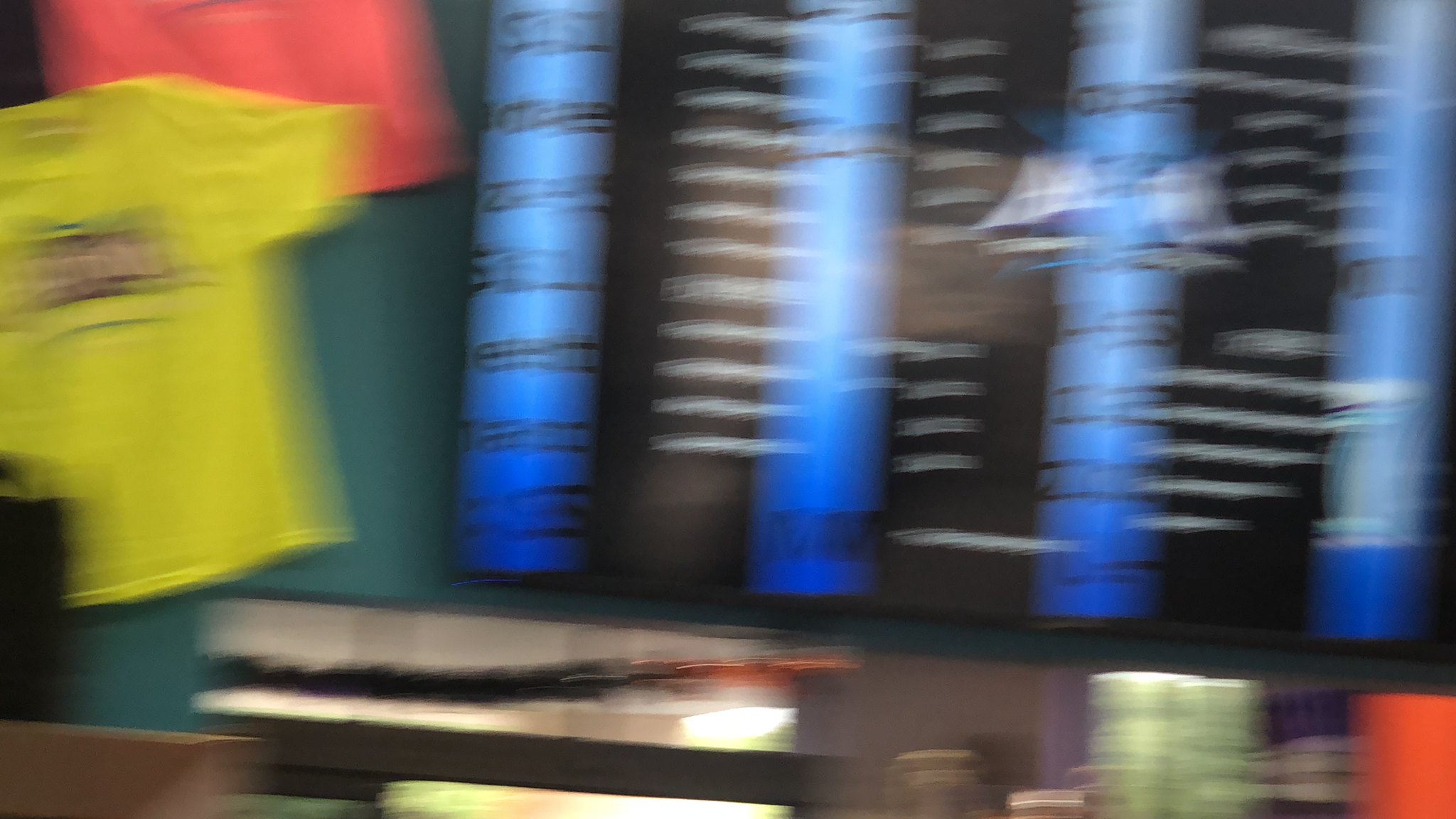The image is a blurry photograph, making it challenging to discern the exact details. On the left side of the image, there are two visible t-shirts—one predominantly yellow and the other a partial view in pink. To the right of the t-shirts, several blue cylindrical shapes descend from the top of the image, which feature some white wording on what might be a blackboard situated between them. The contents of the blackboard are indistinct due to the blurriness but appear similar to a menu board often found in restaurants. Below the cylinders, there are green and red blurry objects that resemble items on a counter, hinting at the possibility of the setting being a restaurant.